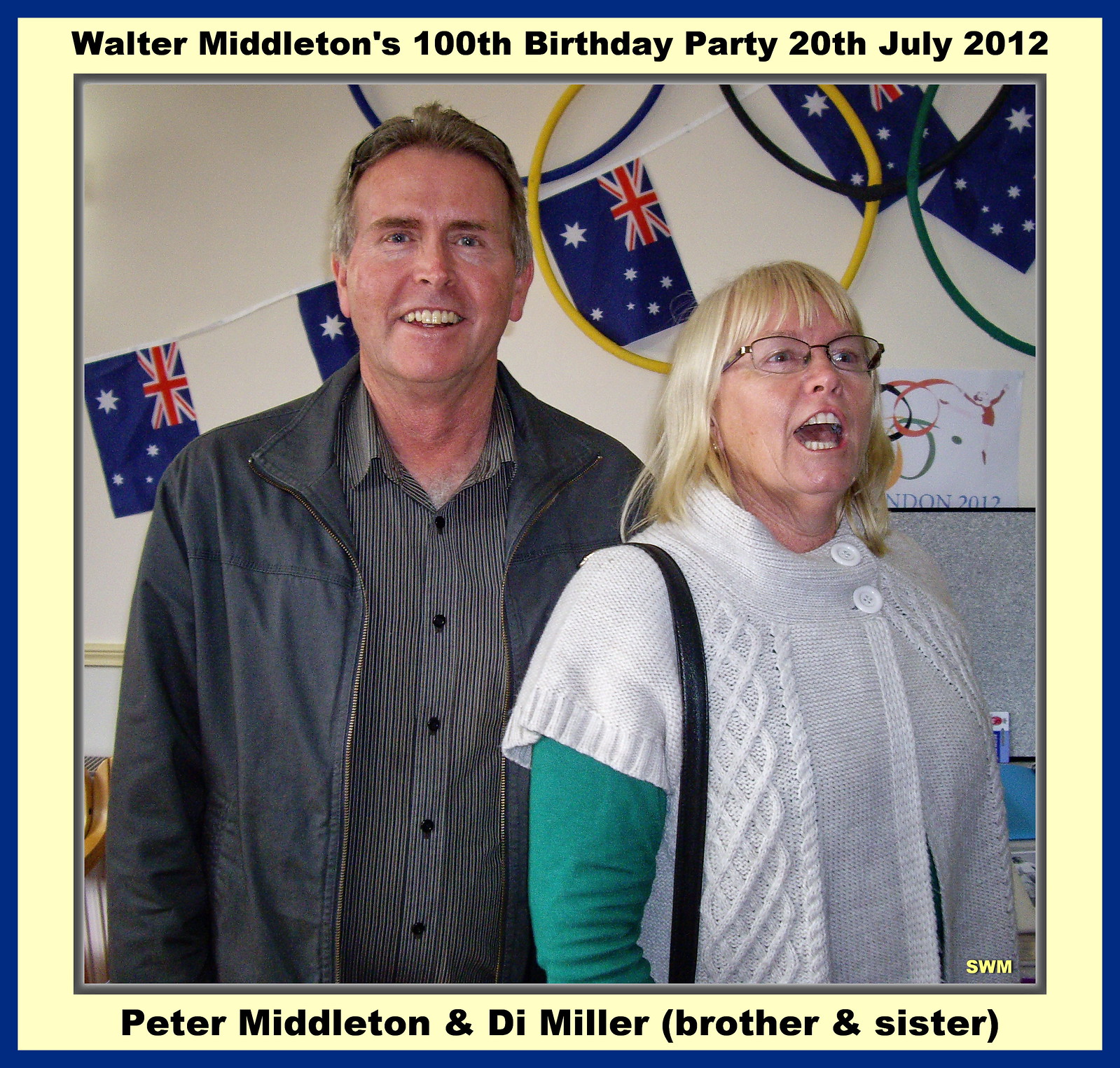In this detailed image, a cheerful man and woman are the central focus against a backdrop of British and Australian flags intermingled with Olympic rings. The man, positioned on the left, dons a light grey jacket over a striped button-down shirt and has short grey hair. He gazes directly at the camera, smiling warmly. To his right stands the woman, engaged in conversation or mid-exclamation, with shoulder-length blonde hair and glasses. She wears a white knitted sweater over an aqua long-sleeved shirt and carries a bag over her right shoulder. The image itself is presented as part of a celebratory card, framed by a blue outer border and a lighter inner frame. Above the photo, the card reads "Walter Middleton's 100th Birthday Party, 20th July 2012," and below it, "Peter Middleton and D.I. Miller (brother and sister)."